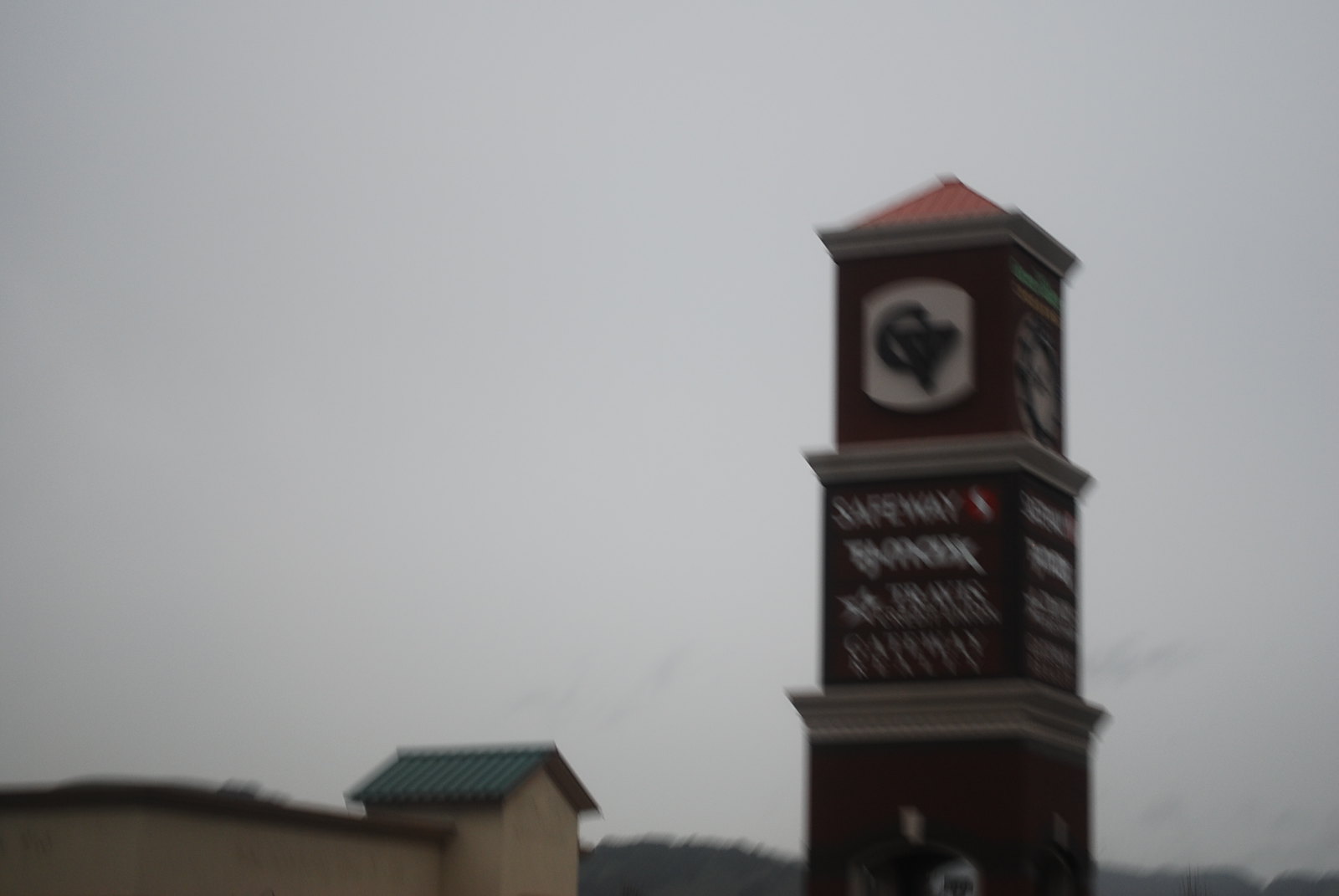In this landscape-oriented, slightly blurry photo, the central focus is a multi-tiered, square-shaped pillar serving as an advertisement for the stores within the shopping center. The discerning store signs visible on the pillar are Safeway and TJ Maxx, while the other store names remain indistinguishable. The pillar is structured with three distinct levels, each separated by trim and slightly smaller in size as they ascend. It is crowned with a pointed, four-sided, pyramid-like top. The base of the pillar is cut off at the bottom edge of the photograph. The background features a gray, overcast sky and the rooftop of one of the shopping center buildings, adding to the suburban commercial atmosphere of the scene.